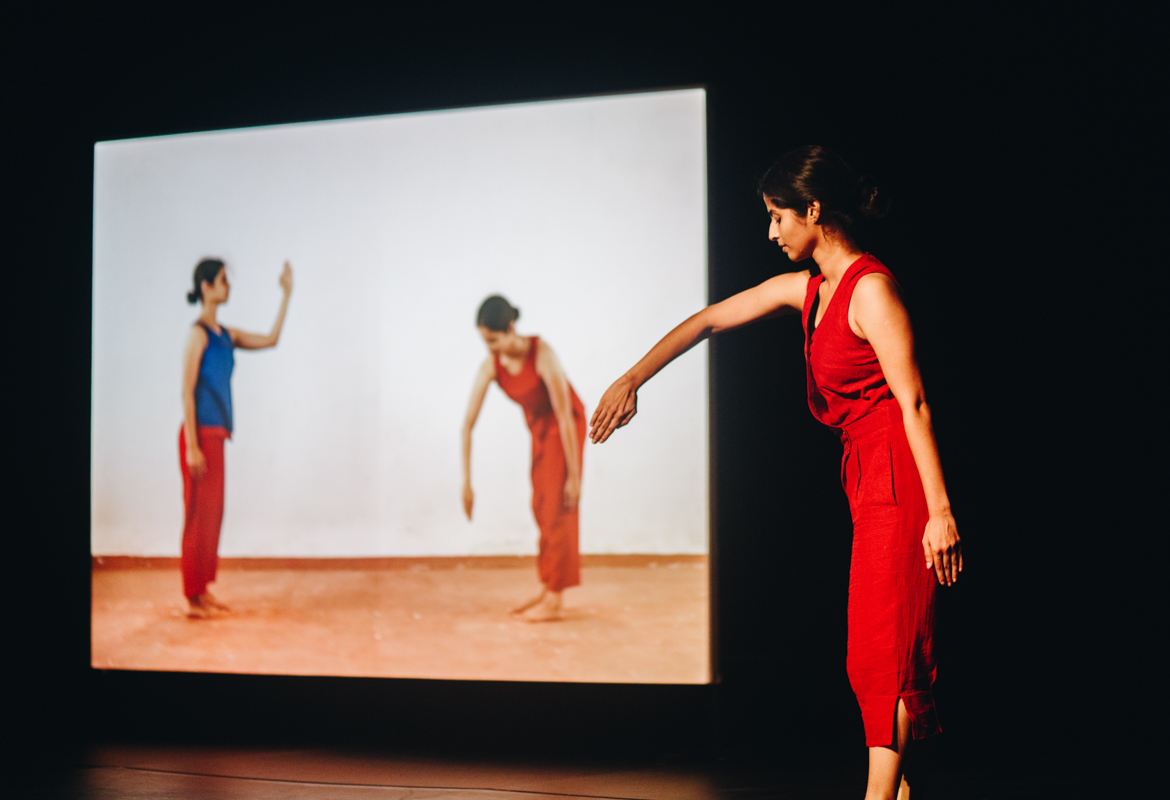In this horizontally rectangular, full-color photograph set against a black background, a woman in a sleeveless red dress stands prominently on the right side. She has dark hair and is posed in profile, her left hand relaxed by her side and her right arm extended forward, gently curved. The red dress goes over her shoulders and extends below her knees. The scene is lit by artificial light and captures an indoor setting with a brown hardwood floor.

To her left, a projection screen displays a digital image featuring two women. One woman, dressed in red like her, is bent over with her arms hanging down, mirroring the pose of the woman standing nearby. Next to her on the screen is another woman wearing red pants and a blue blouse, standing with her right hand at her side and her left hand raised at a 90-degree angle. Both women in the digital image are barefoot, suggesting a display of dance, gymnastics, or exercise technique. The woman standing in red appears to be visually demonstrating the poses shown on the projection screen.